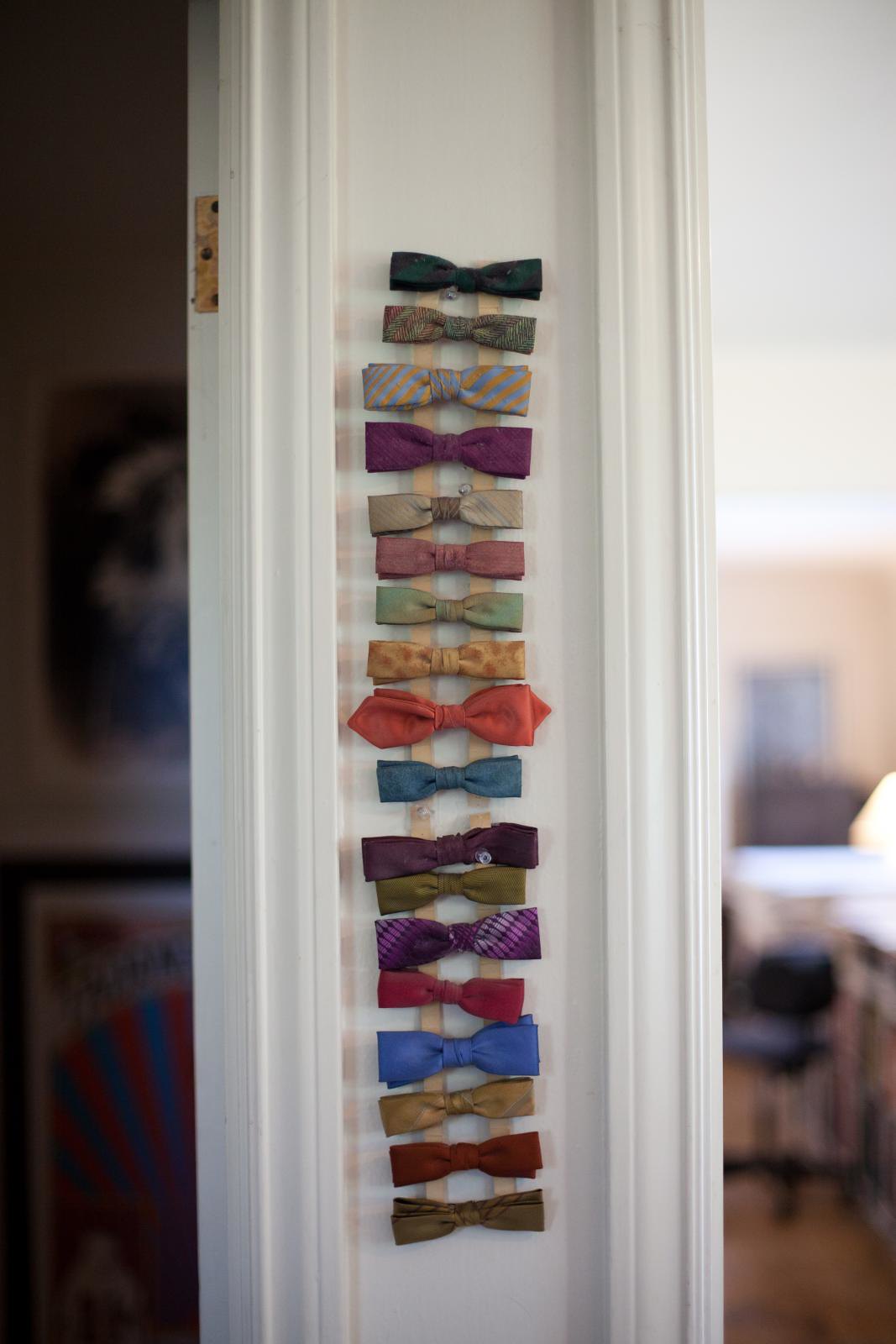The photograph captures a section of a white wall divider between two door frames, adorned with a meticulously arranged wall hanging of 18 vibrant bow ties. These bow ties are of various colors and designs, including solid shades of blue, red, purple, orange, pink, and green, alongside patterns like stripes and plaids. The bow ties, which are each large enough to be clip-on accessories for men, are neatly stacked vertically with small gaps between them, attached to two ribbons that hang down the wall, held in place by a thumbtack. The scene offers a glimpse into an adjacent room that is lit, featuring a bar stool, a countertop, and an illuminated lamp, adding a cozy ambiance to the meticulous display of bow ties on the white, molded divider wall.